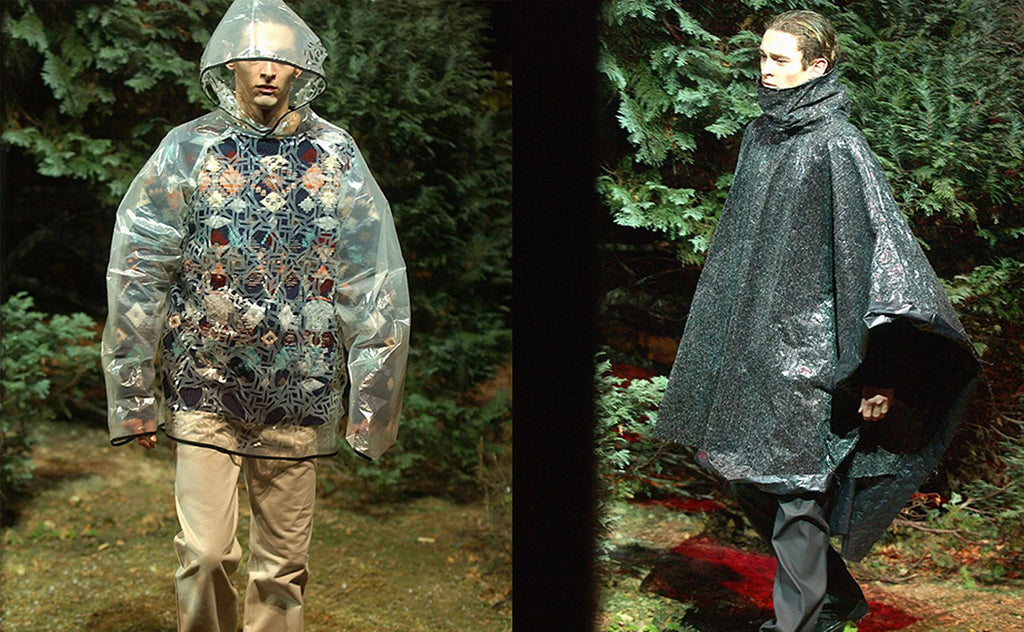This image features two color photographs placed side by side, separated by a thick black divider, each depicting a model in a rain slicker. The left photograph shows a person, who could be perceived as either a man or woman, wearing a clear, slightly transparent rain slicker with an oversized hoodie. Underneath the slicker is a multicolored, long-sleeved knit sweater adorned with varied patterns, predominantly in browns, tans, and blues. The model is also dressed in khaki pants, standing against a backdrop of bushes that hint at an outdoor setting, possibly suggesting these are advertisement shots for rainwear.

The right photograph captures the same individual in a different rain slicker, this time a gray, poncho-style plastic rain jacket. This jacket features a large cowl neck that billows out behind them. The model’s gray pants complement the jacket, and they stand against a similar nature-inspired background with trees and a gravel road, continuing the outdoor theme.